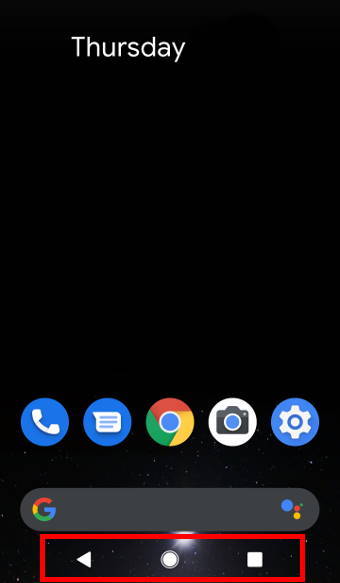In this detailed screenshot set against a black background, we're observing a vertically elongated image with several distinct elements. At the very top, the word "Thursday" is prominently displayed in white text. Moving down to the bottom third of the screen, we encounter a row of various application icons. From left to right, these icons include:

1. A blue circle featuring a white bone,
2. A messaging app icon within a blue circle,
3. The Google Chrome icon,
4. A camera icon encased in a gray circle,
5. A blue circle with a white settings gear.

Directly below this row is a dark gray box. On the left side of this box is the letter 'G' representing Google, while on the right side, there are small circles in Google’s signature colors — red, blue, yellow, and green.

Finally, at the bottom of the screenshot, there are three navigation icons outlined with a thin red border:

1. A left-pointing arrow on the left,
2. A central home button in the shape of a circle,
3. A square white icon on the right, presumably representing the recent apps or multitasking feature.